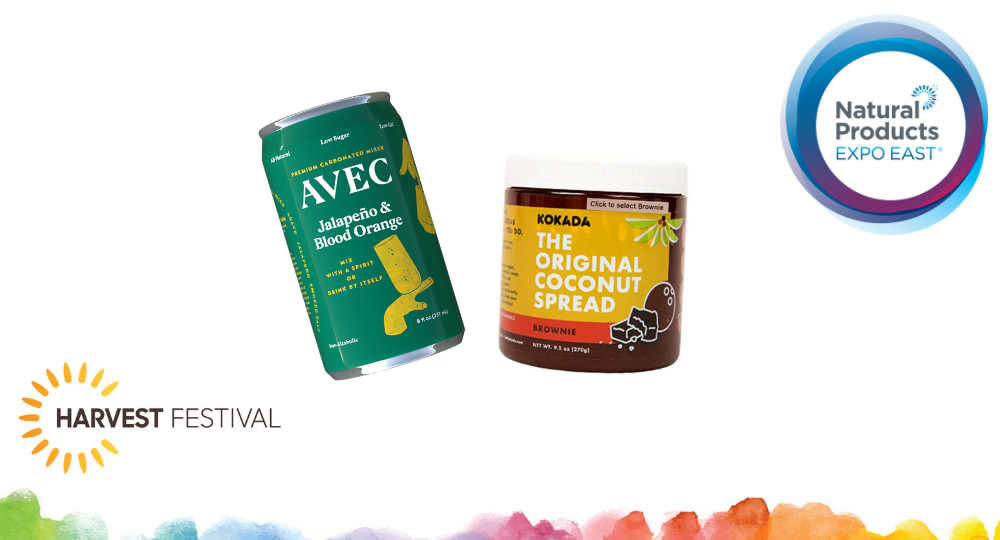This advertisement for the Harvest Festival features significant white space with a vibrant watercolor wash border along the bottom, transitioning through green, blue, purple, berry, orangey red, and yellow hues. In the bottom left corner, the Harvest Festival logo, resembling the sun with gradient orange dashes, accompanies the words "Harvest Festival" in bold and light fonts. Centrally displayed are two products: a green beverage can labeled "Avec Jalapeno and Blood Orange," promoting itself as a "Premium Carbonated Mixer" suitable for mixing with spirits or drinking alone, and a jar with a white lid and a brown bottom labeled "Cocotta The Original Coconut Spread Brownie," featuring a yellow and red label with cocoa bean illustrations. The top right corner displays a circular logo in various shades of blue and ruby, stating "Natural Products Expo East." The overall lighting of the image is bright and modern.